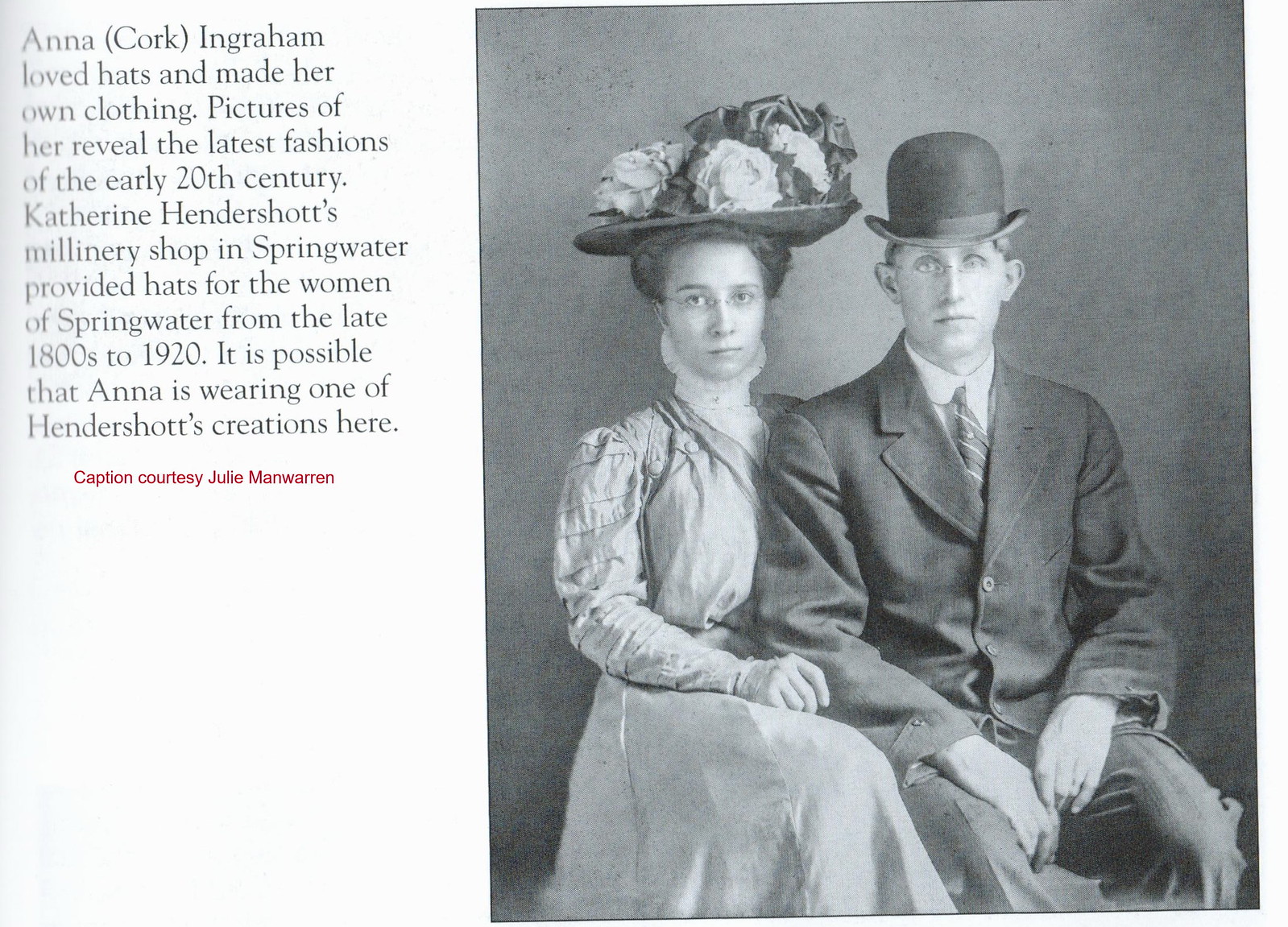This black-and-white photo, situated on the right side of the page, features a seated man and woman dressed in early 1900s attire. The woman, positioned on the left, wears glasses and a large brimmed hat adorned with flowers. Her outfit includes a lace-like turtleneck and a long dress. The man to her right sports a hat with an upturned brim, glasses, a dark suit, a button-up shirt, and a tie. The text on the left side of the page reads: "Anna Cork Ingraham loved hats and made her own clothing. Pictures of her reveal the latest fashions of the early 20th century. Catherine Hendershott's millinery shop in Springwater provided hats for the women of Springwater from the late 1800s to 1920. It is possible that Anna is wearing one of Hendershott's creations here." The caption is credited in red text at the bottom, stating, "Caption Courtesy Julie Manwarren."